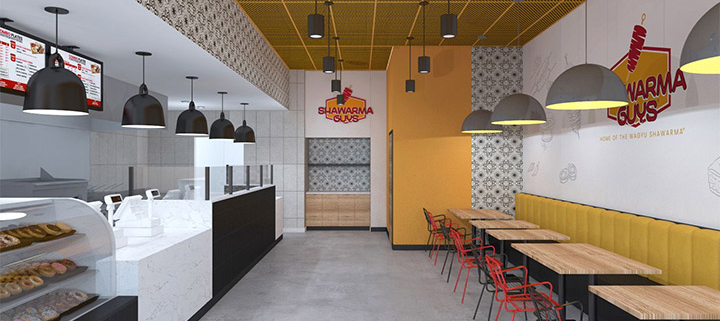This photo, taken from inside a restaurant named "Shwarma Guys," captures a detailed view of its interior. The shot is aligned parallel to a white countertop on the left side, where food is prepared and served, separated by a glass divider. Below this countertop, there is a display case showcasing an assortment of donuts and pastries. Above the countertop, black metal pendant lights hang from the brown wooden lattice ceiling, illuminating the food line and the cashier area. 

The restaurant features a concrete gray floor and diverse wall treatments. The right side wall is primarily white, adorned with a red and orange "Shwarma Guys" logo, while the far right corner includes a yellow section. The walls also incorporate green and black geometric patterned wallpaper, seen both in the upper right corner and the back, extending above the countertop where the main operations occur. 

The seating area on the right comprises a long booth with a yellow back and black seats, flanked by light wooden tables. Metal chairs, red and black in color, add to the eclectic seating arrangement. Above the tables, additional black pendant lights hang. Further back, a menu board with white background and black, red, and yellow text can be seen, though the text details are indistinguishable due to distance. The overall ambiance of "Shwarma Guys" combines modern elements with a warm and inviting aesthetic, highlighted by its colorful and varied decor.